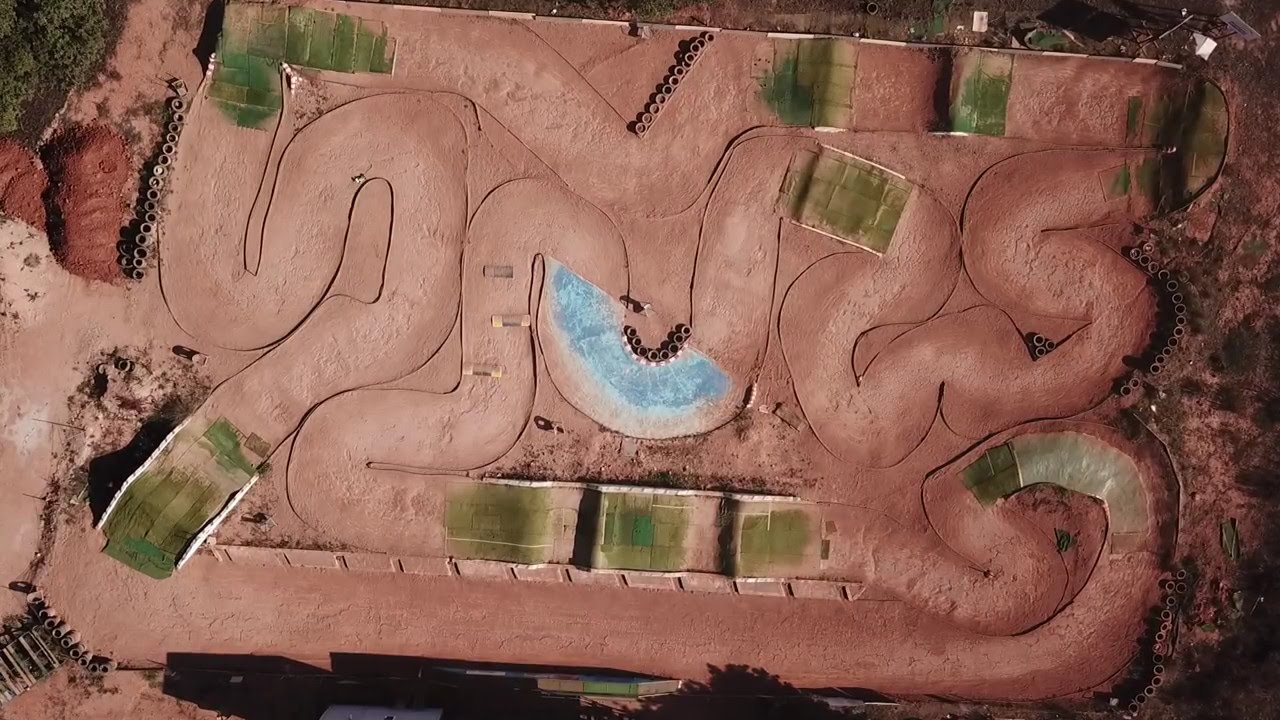The landscape-oriented color photograph, likely captured by a drone, presents a top-down view of what appears to be a construction site resembling a labyrinthine water park. The scene is dominated by a reddish-brown, rectangular expanse of dirt interspersed with a series of undulating, snake-like paths. These winding sections exhibit a rust-red hue, suggesting they might be made from rock or plaster. In the center of one of these curves, a light blue feature, possibly a water element or a semi-filled drain, catches the eye. The image includes patches of green grass in the bottom left, top left, and top right corners, adding a touch of color contrast to the predominantly earthy tones. Towards the bottom, three light-colored squares with a smeary mix of green and brown are visible, potentially indicating areas under development. The upper left corner of the image reveals a large section of stacked pipes, hinting at ongoing infrastructure work. The photograph exemplifies a style of photographic realism, emphasizing the intricate details and textures of the construction site's layout.